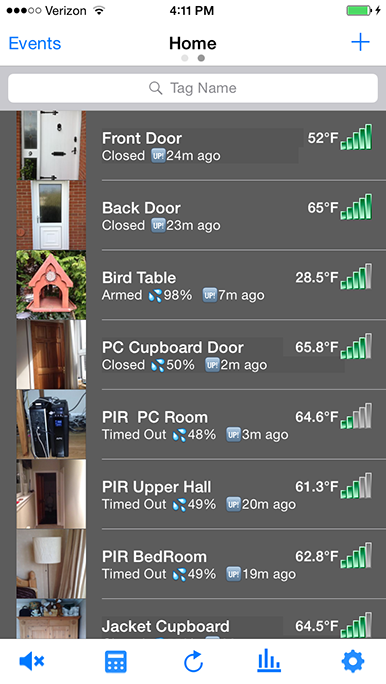A detailed caption for the image:

---

The image displays an interface serviced by Verizon, capturing real-time data from various smart devices integrated into a home. The screen showcases logged events from devices connected to doors, rooms, and specific areas within the home, accessible through a software application on a phone, tablet, or computer. The detailed log includes:

- **Front Door**: Closed 24 minutes ago, temperature at 52°F.
- **Back Door**: Closed 23 minutes ago, temperature at 65°F.
- **Bird Table**: Armed 70 minutes ago, temperature at 28.5°F.
- **PC Cupboard Door**: Closed 2 minutes ago, temperature at 65.8°F.
- **PIR (Passive Infrared) PC Room**: Accessed 3 minutes ago, temperature at 64.6°F, with a bar graph indicating 2-3 bars of activity.
- **PIR Upper Hall**: Accessed 20 minutes ago, temperature at 61.3°F, with a bar graph indicating 2-3 bars of activity.
- **PIR Bedroom**: Accessed 19 minutes ago, temperature at 62.8°F.
- **Jacket Cupboard**: The detailed data isn't entirely visible, but it shows a temperature of 64.5°F.

The interface also includes temperature readings for each device with bar graphs indicating the activity level, with most bars in the range of 4 to 5 bars full, except for the PIR PC Room and PIR Upper Hall, which show 2 to 3 bars.

---